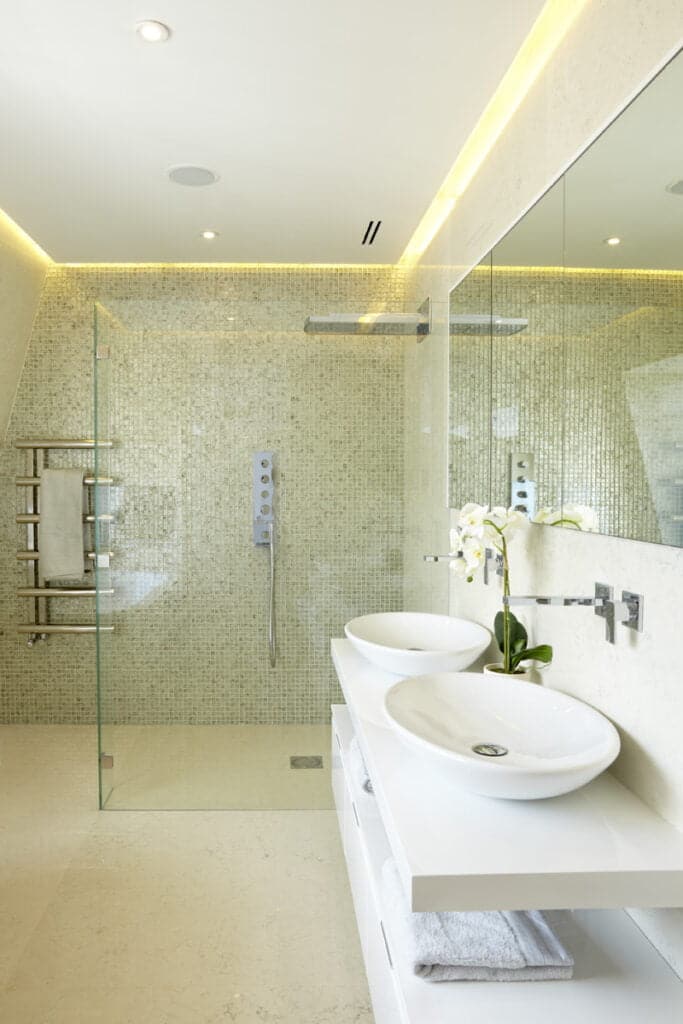This image showcases a beautifully renovated, modern bathroom with a sleek, Asian-inspired design. The entire space exudes elegance with its light palette of whites and tans. In the foreground on the right side, there is a double sink setup featuring two raised white porcelain basins positioned on top of a white hanging shelf. A delicate white orchid sits between the basins, adding a touch of natural beauty. Behind the sinks, a three-panel glass mirror spans the wall, providing a sense of depth and space.

Towards the back of the image, a standing shower occupies the distance, seamlessly integrated with the rest of the bathroom through the use of a clear glass partition. The shower area, distinct yet connected, features a large, protruding metal shower head and additional shower nozzles on the side, set against intricately tiled walls in varying shades of tan.

To the left of the shower, a thick, golden-colored metal towel rack stands out, offering both functionality and a hint of luxury. Above, the ceiling's edges are adorned with a light strip, casting a soft golden glow throughout the room. The entire scene is cohesive, modern, and elegantly styled, reflecting meticulous attention to detail and contemporary aesthetics.